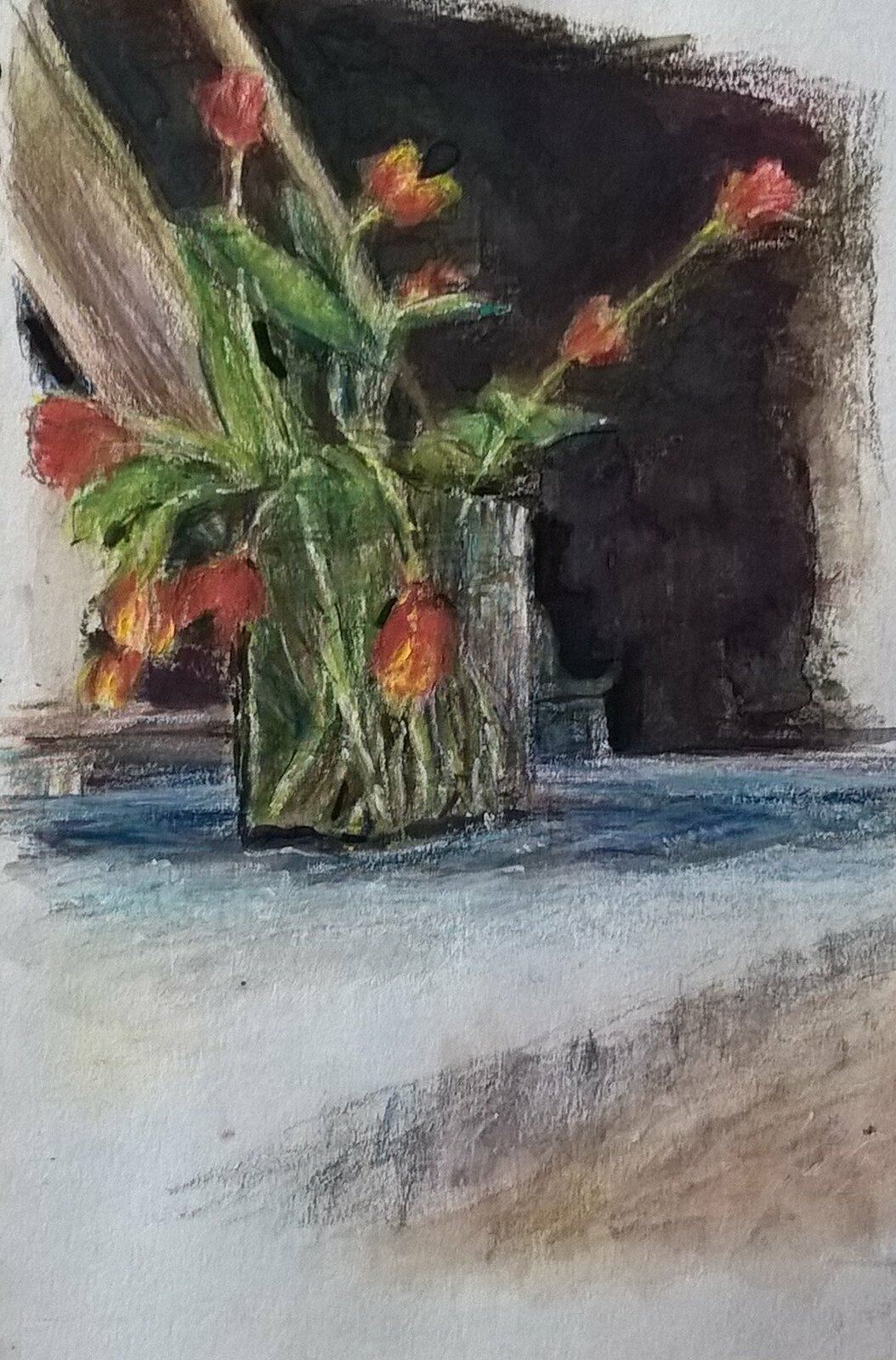The image is a detailed painting of vibrant flowers arranged in a clear glass vase, through which their green stems and leaves are visible. The flowers, predominantly red with hints of yellow, are in various stages of bloom; some are fully blossomed while others remain closed. Several flowers are wilted, their stems bent gracefully over the sides of the vase. The glass vase appears to be slightly overflowing, with blue droplets of water spilling onto the brown table beneath. The table, extending to the bottom of the image, has subtle shades of blue, brown, white, and black, adding depth and texture. The background is predominantly brown with some shadowing to enhance depth, and includes what seems to be a wooden beam on the left side, adding a rustic touch to the overall composition.